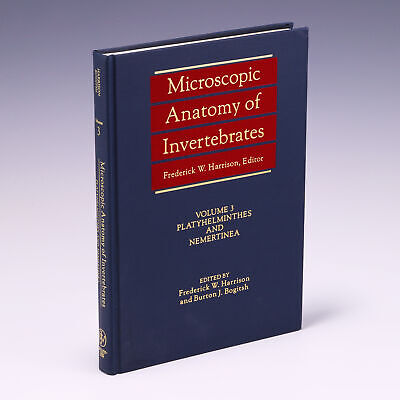The photograph showcases a dark blue hardcover book titled "Microscopic Anatomy of Invertebrates," prominently displayed in gold text. Each word of the title is separated by a red rectangle with slight spacing in between. Below the title, in gold text, it reads "Volume 3, Platyhelminthes and Nemertinea," and further beneath, "Edited by Frederick W. Harrison and Burton J. Bogitsh." The spine, also visible, carries the book's title in gold text. The book is set on a gradient background transitioning from dark purple at the top to light purple at the bottom.